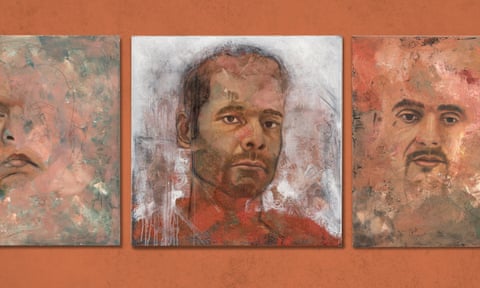Set against a burnt orange, rusty background, this photograph captures three square canvas paintings in a row, each presenting a semi-abstract portrayal of men's faces. The leftmost canvas is slightly cut off in the image, revealing only the lips, one nostril, and part of an eye of a man. This painting features an abstract mix of pink (resembling Pepto-Bismol) and green, with accents of gray and white around the edges. The center canvas is more defined, showing a man with a goatee, a short beard, and dressed in a red jacket. The man's face is more wholly depicted against a background of white, gray, and red hues, with the facial details clearly visible. The rightmost canvas displays a man's face prominently set against a background of red, brown, tan, and pink abstract shades. Here, the man has deep-set eyes, thick brown eyebrows, thin lips, and a brown goatee, but his hairline, head, and neck are not visible. All three paintings present a compelling blend of color and form, each contributing uniquely to the semi-abstract ensemble.